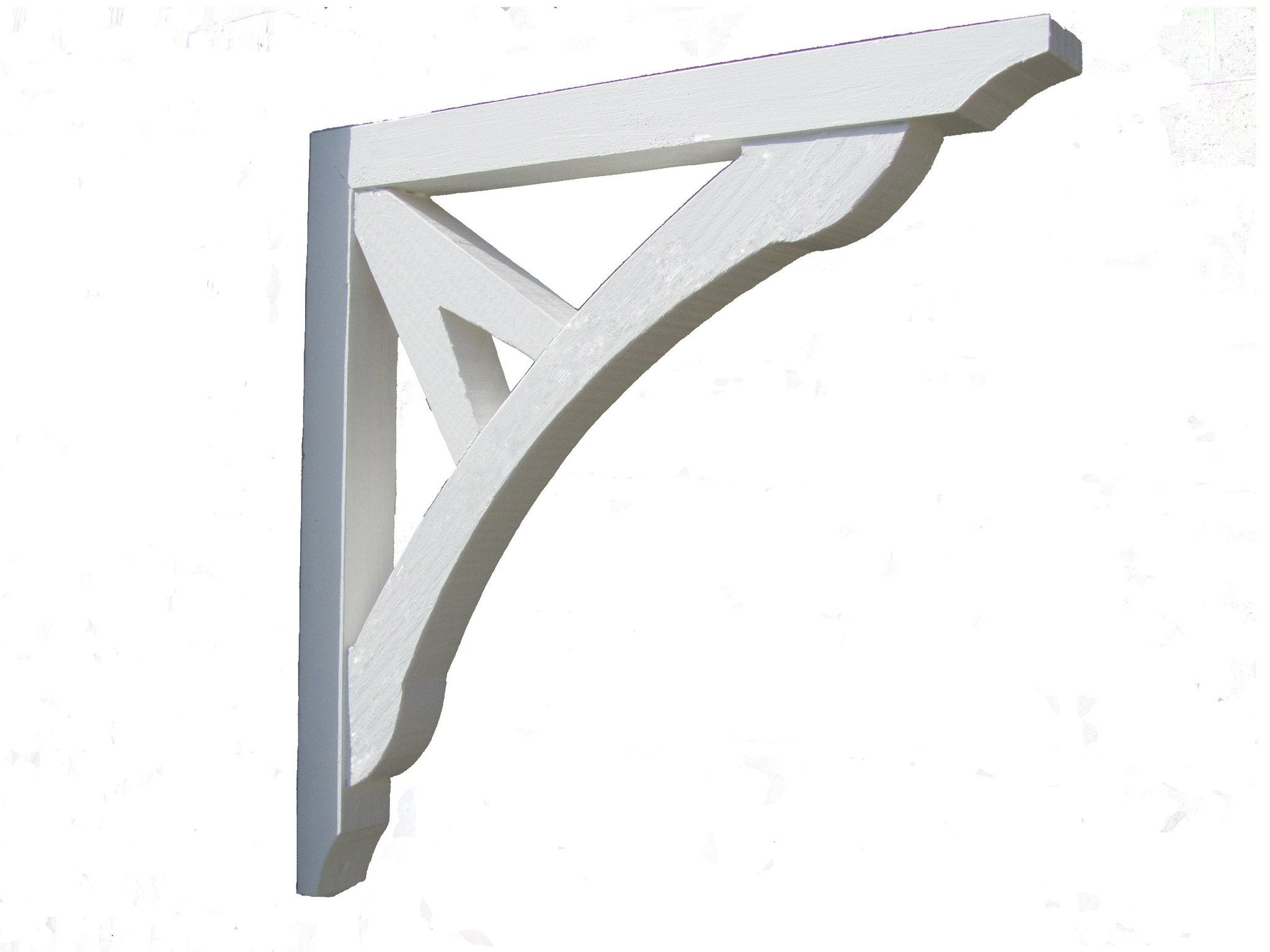The photograph features a distinctive decorative wall bracket designed for corner placement. The main structure consists of a perfect triangular framework with a unique combination of white and gray elements. On the left side, there's a vertical gray bar attached to a horizontal white bar at the top, creating a supportive structure. Connecting these bars is a curved white piece and two smaller pieces forming an 'A' shape, adding to the design's complexity. This triangular bracket, primarily white with potential metallic hints, appears to serve both decorative and functional purposes, such as supporting a shelf or accentuating a room's corner. The background of the photograph is plain, ensuring the focus remains on this intriguing wall décor.